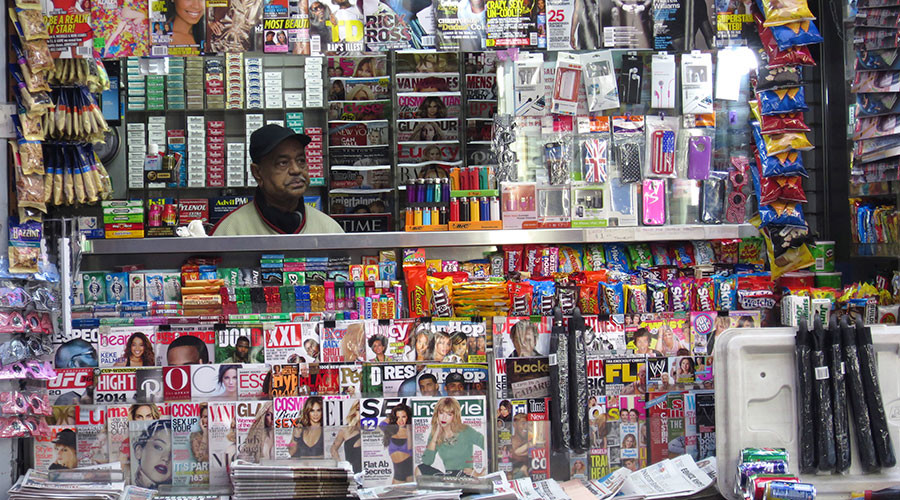In this image set inside a bustling convenience store, the visually crowded scene features a diverse array of merchandise covering nearly every inch. The lower part of the image showcases rows of various magazines, including titles like Cosmo, InStyle, and XXL. Above the magazines, shelves brimming with candy display brands such as Reese's, M&M's, and Skittles. Toward the right, bags of chips are visible.

Central to the image is an older African-American man seated behind the counter, wearing a black cap, a gray jacket with red stripes down the shoulder and a red collar, and headphones around his neck. Behind him, a shelf is stocked with cigarette packs, including Marlboro, and additional racks hold phone cases and lighters.

On the counter and surrounding shelves, an overflow of items like peanuts and gum adds to the cluttered yet well-stocked atmosphere typical of a convenience store. Despite the abundance of objects and colors—ranging from red, white, green, purple, black, pink, tan, blue, orange, and yellow—there is a notable lack of readable text beyond the product packaging and magazine covers. The man appears to be looking out, possibly awaiting a customer, in this vibrant and busy indoor setting.